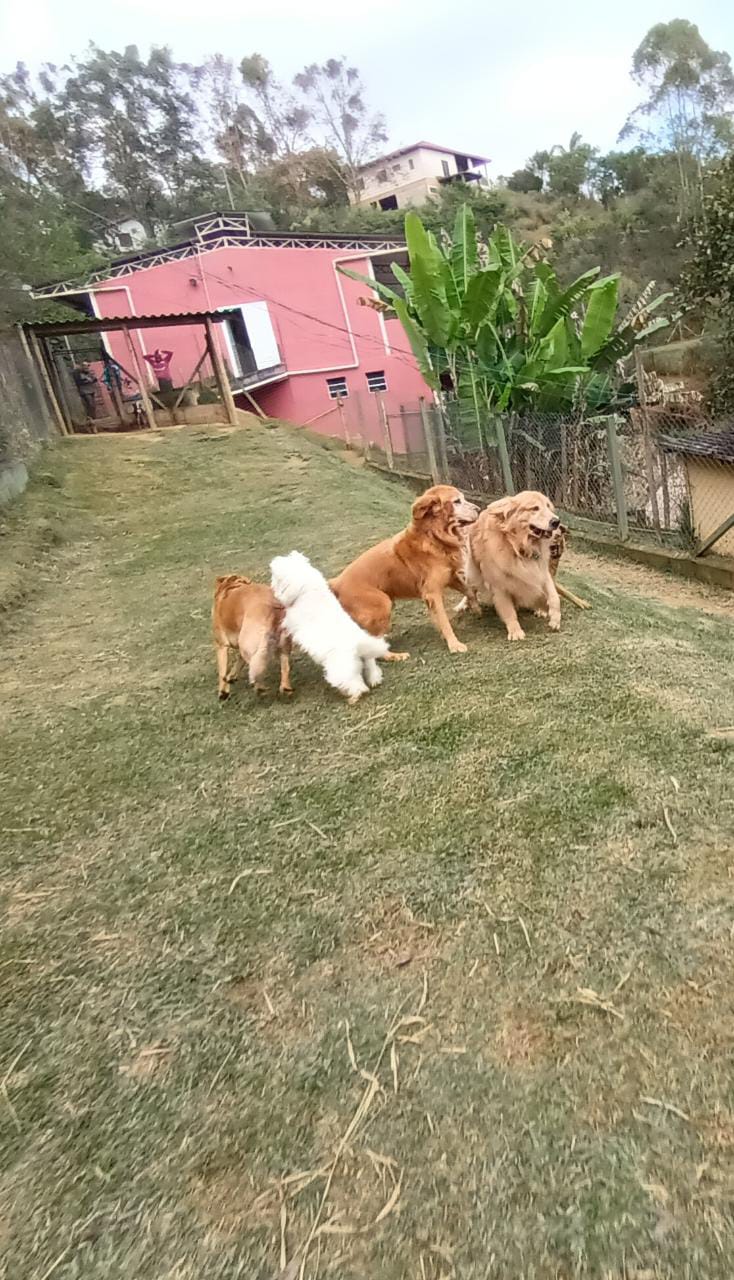The image features a vibrant scene of four dogs in a yard with short grass. Two golden retrievers are positioned toward the bottom right of the image, seeming to observe the activity, while a small white dog and a light brown dog frolic towards the top left. The dogs are captured from various angles, including both back and side views. Behind them, a person stands watching the playful canines. Dominating the background is a quaint pink house with a white door, partially shielded by a tall green plant. Further in the distance, a white house perches on a hill, framed by a bright blue sky and a scattering of trees. The yard's lively ambiance is accentuated by the mix of dog breeds and sizes, bringing warmth to the scenic household view.